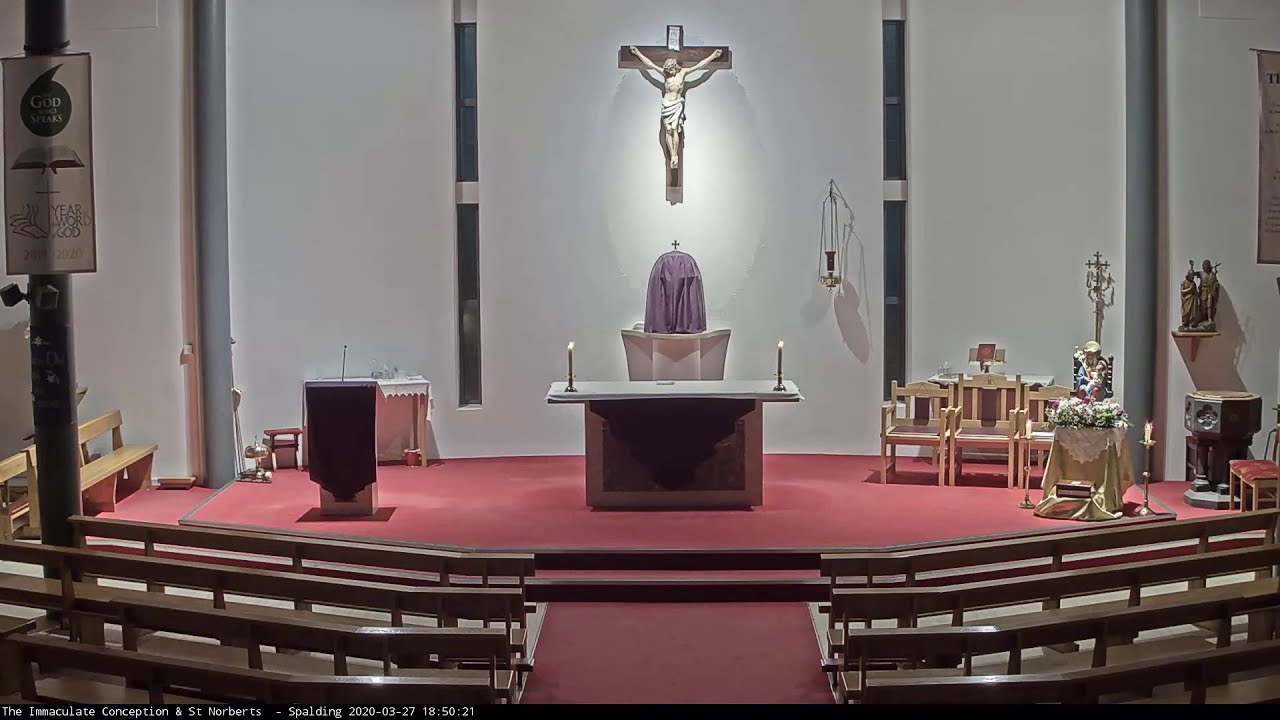The image depicts the interior of a Catholic church, focusing on a prominently situated altar area. Dominating the center of the scene is a large crucifix of Jesus Christ, affixed to a white wall behind the altar. Beneath the crucifix, an altar draped with a purple cloth covers a podium, and a small cross rests atop this cloth. Flanking the altar are two lit candles, providing a serene illumination. The floor leading up to the altar is covered with a thin red carpet, and two steps ascend to this sacred space.

On the left side of the altar, there are three white wooden chairs and a smaller pulpit adorned with a microphone. To the right, additional chairs and statues are positioned, their details less discernible. Further left, a pole displays a banner picturing an open Bible and the words, "Year, Word, God."

In front, there are several long white bench pews for congregants, arranged in rows and extending out toward the viewer's standpoint. The area appears well-lit, enhancing the reverent and peaceful atmosphere characteristic of a place of worship. A small, unreadable sign in the background at the bottom of the image states "Immaculate Conception."